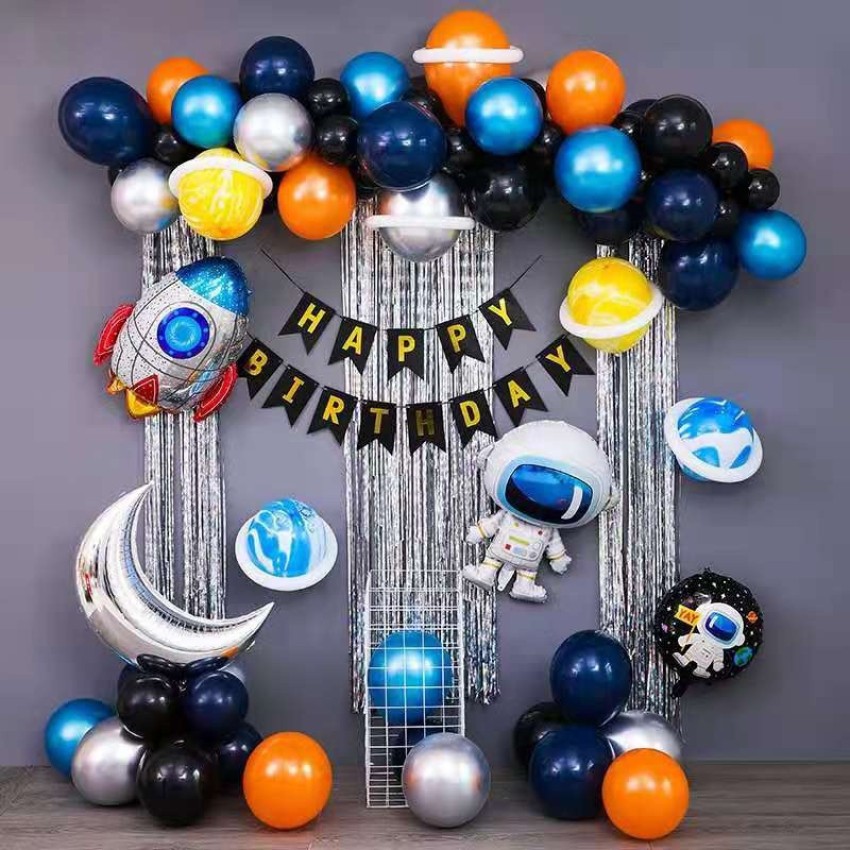The image showcases an elaborately decorated gray wall celebrating a birthday with a space-themed motif. Dominating the upper section is a vibrant balloon arch that features an array of colors: orange, light blue, dark blue, black, silver, and yellow. Many of these balloons are creatively styled to resemble planets, with some adorned with white rings to mimic the look of Saturn. Among these planetary balloons is a striking silver balloon with a white ring as well. The highlight of the decor is a black and gold "Happy Birthday" banner prominently displayed at the center.

Adding to the cosmic ambiance, a variety of themed balloons and decorations further enhance the scene. To the left of the banner, a colorful rocket ship balloon, featuring red, blue, silver, and orange hues, is positioned for liftoff. Below the banner, an astronaut balloon appears as if it is floating in space. Several blue planet-like balloons with a marbleized appearance are strategically placed on the wall. Near the bottom, a silver crescent moon balloon rests closer to the ground amidst an assortment of additional balloons in dark blue, orange, silver, and light blue.

Complementing these elements, an arrangement of metallic streamers, possibly silver tassels, hang down creating a dynamic backdrop. Small plush toys, including the astronaut and other space-themed elements, add a whimsical touch, completing this atmospheric and playful birthday display.